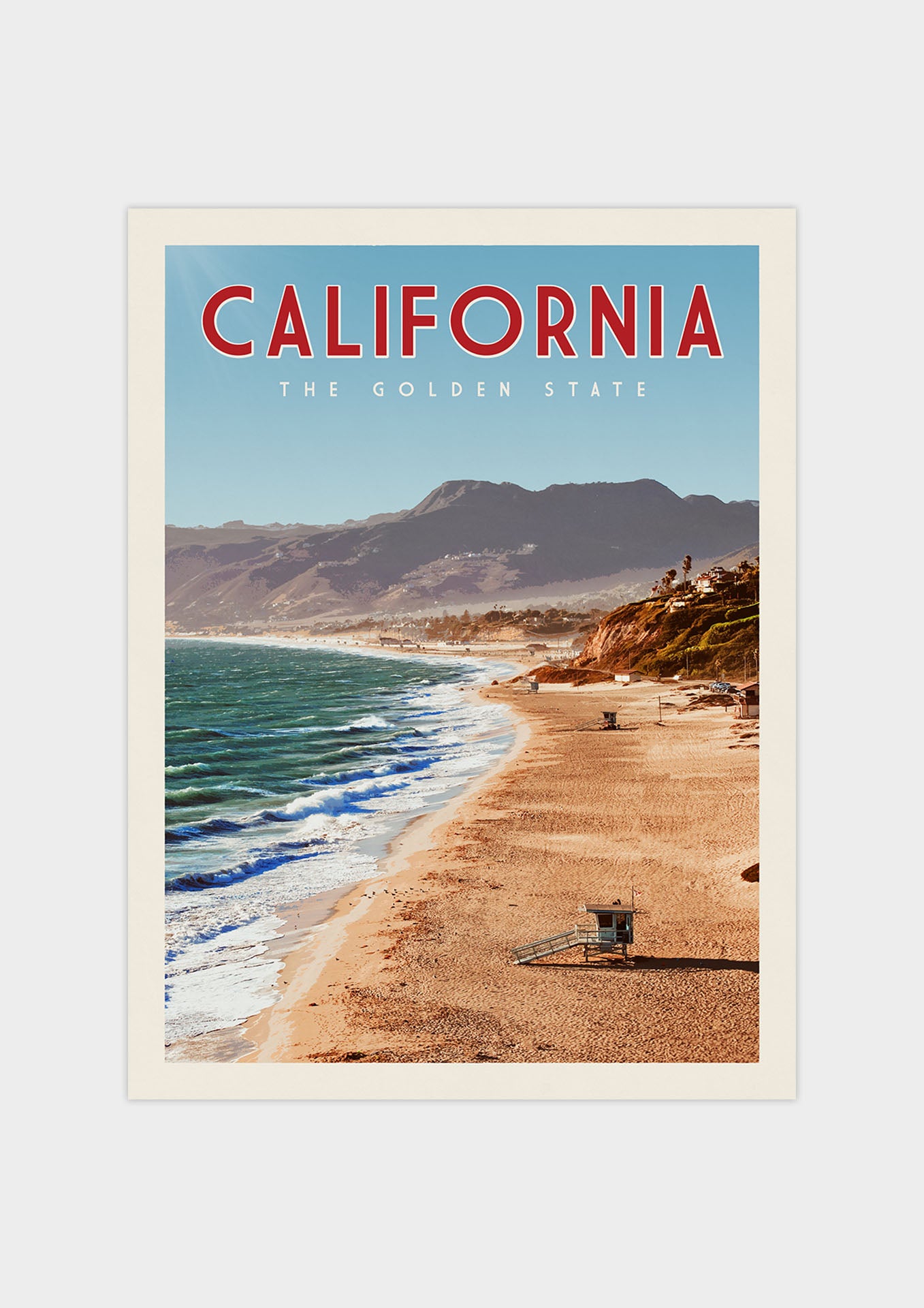This image is a small photo of a California beach scene, printed on a white piece of paper. The photo has a thin white border, clearly distinguishable from the white background it rests on, as if mimicking a framed picture hanging on a wall. At the top of the photo, in bold red letters, it reads “California,” with a white outline. Beneath it, in smaller bold white letters, it says "The Golden State."

The photo captures a long stretch of a classic, tan-colored sandy beach on the right side. Prominent in this area are a couple of lifeguard houses, elevated on stilts with long staircases extending from the front. The left side of the image reveals the choppy, green water of the ocean, with white foamy waves crashing energetically against the shore. In the distance, towering over the scene, are steep, rocky cliffs in a brown hue, adding a rugged backdrop to the serene shore. Above the cliffs, a light blue sky completes the picturesque California beach scene.